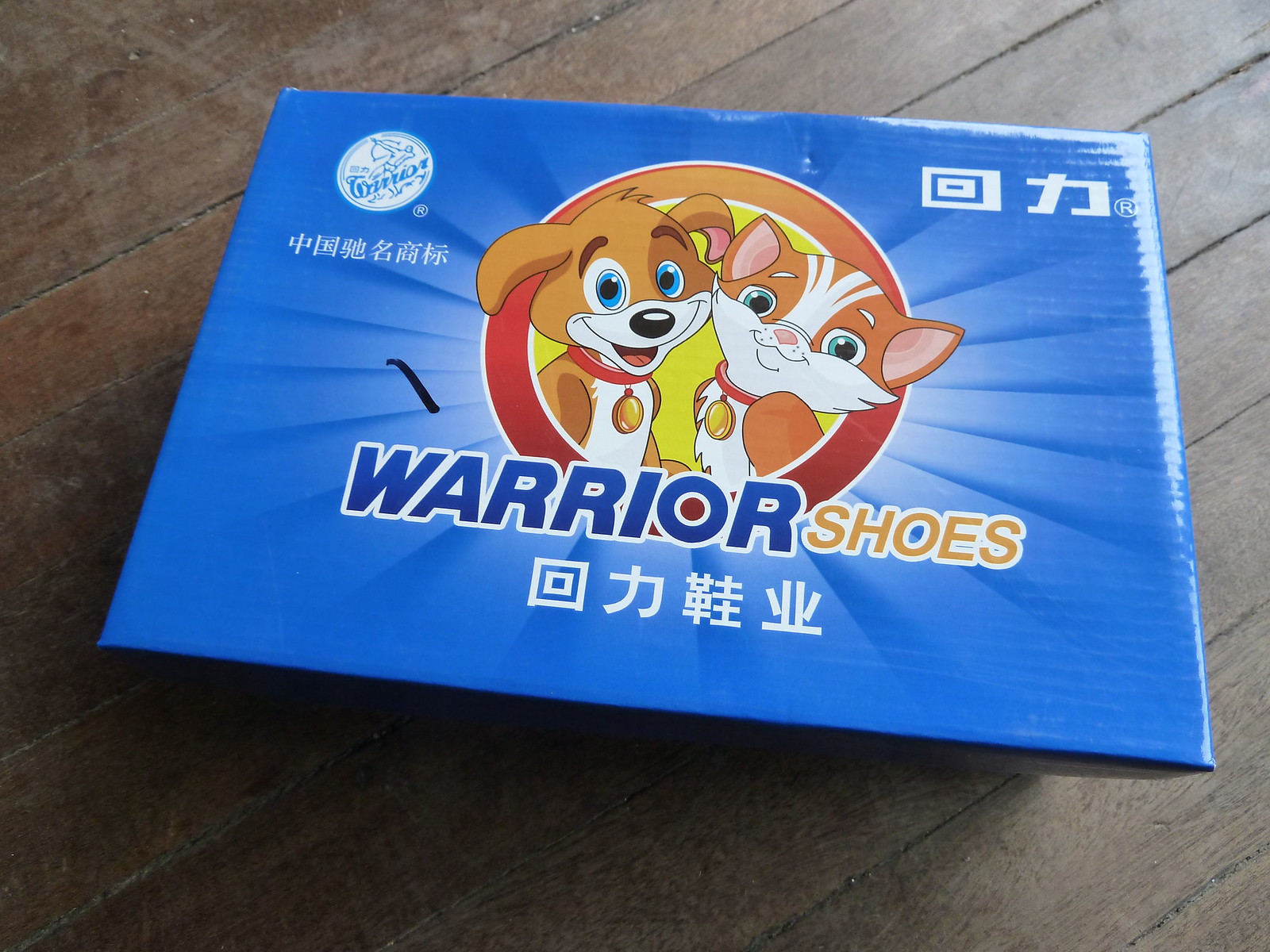This image is a photograph depicting the top of a rectangular, bright blue cardboard shoebox sitting on a dark wood grain slatted tabletop. The center of the box features a cartoonish illustration within an orange circle, showing a brown puppy with blue eyes and a red collar with a gold medallion, alongside an orange kitten with green eyes, also wearing a red collar and a gold medallion. Both animals appear to be smiling. Above them, the text "Warrior Shoes" is prominently displayed, with "Warrior" in blue and "Shoes" in gold, and beneath it, there are four characters in an Asian language. In the top left corner of the box, there is another logo with the word "Warrior" and additional unfamiliar characters underneath. The top right corner features two more Asian characters alongside a registered trademark symbol.